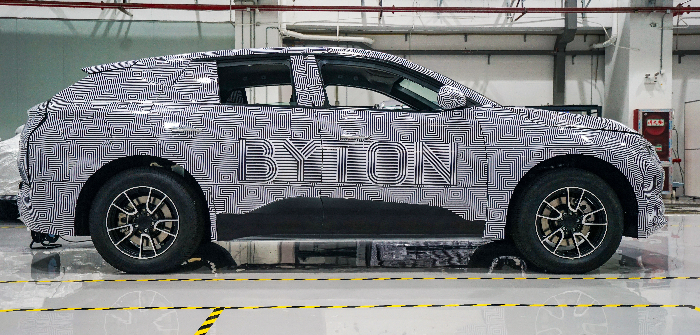This detailed image captures a car parked in a factory setting, showcasing a unique and eye-catching custom wrap. The car displays a geometric, black-and-white maze-like print that spans across the entire body, giving it an overall gray appearance. Prominently displayed on the right side of the car, stretching from the back door to the front door, is the name "BYTON" rendered in intricate line-based lettering. Below this, there is a black sloping section at the bottom of the doors.

The car is positioned on a highly reflective, light gray floor, which mirrors the vehicle due to the lighting within the facility. The floor features distinct yellow and black striped tape markings that hint at lanes or safety zones. The factory background includes a green wall to the left and white or gray walls to the right, with a visible pipe running across the walls. Additionally, there is a door to the right with some sort of adjacent machine, possibly for air management. This vividly detailed photograph, captured in landscape orientation, embodies photographic realism.